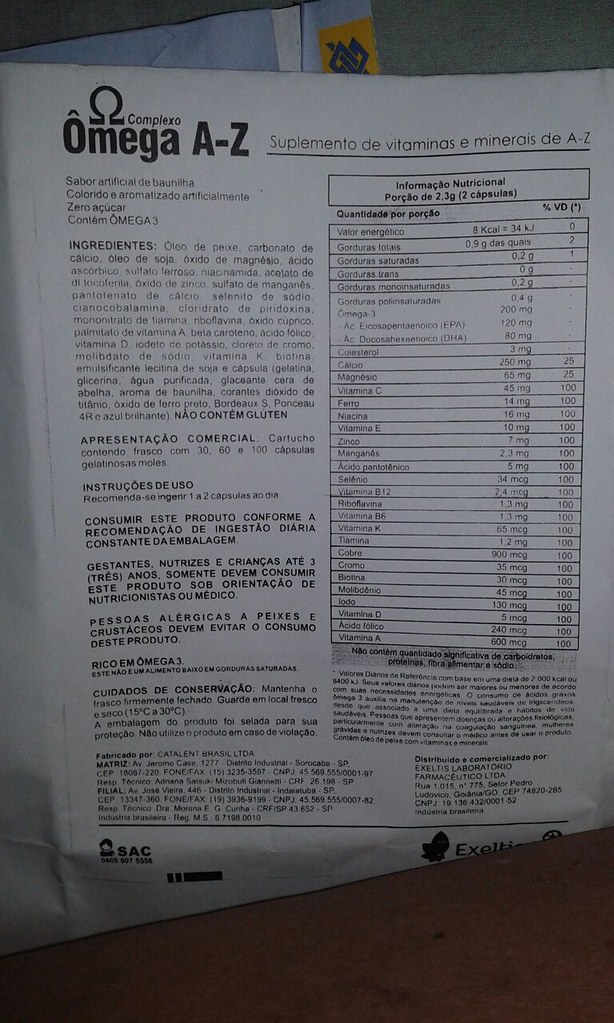The vertical rectangular image predominantly showcases the nutritional information of a product, likely a dietary supplement, with details in Portuguese. At the top, it prominently features the product name, "Complexo Ômega A-Z", followed by a description stating "Suplemento de Vitaminas e Minerais A-Z." The entire packaging is in white and adorned with black text. Centrally placed is a table that outlines the nutrition facts, including various vitamins and their respective daily percentage values, all enclosed within a black border. At the bottom of the image, there is text detailing the product's origins, indicating it is manufactured in Brazil.